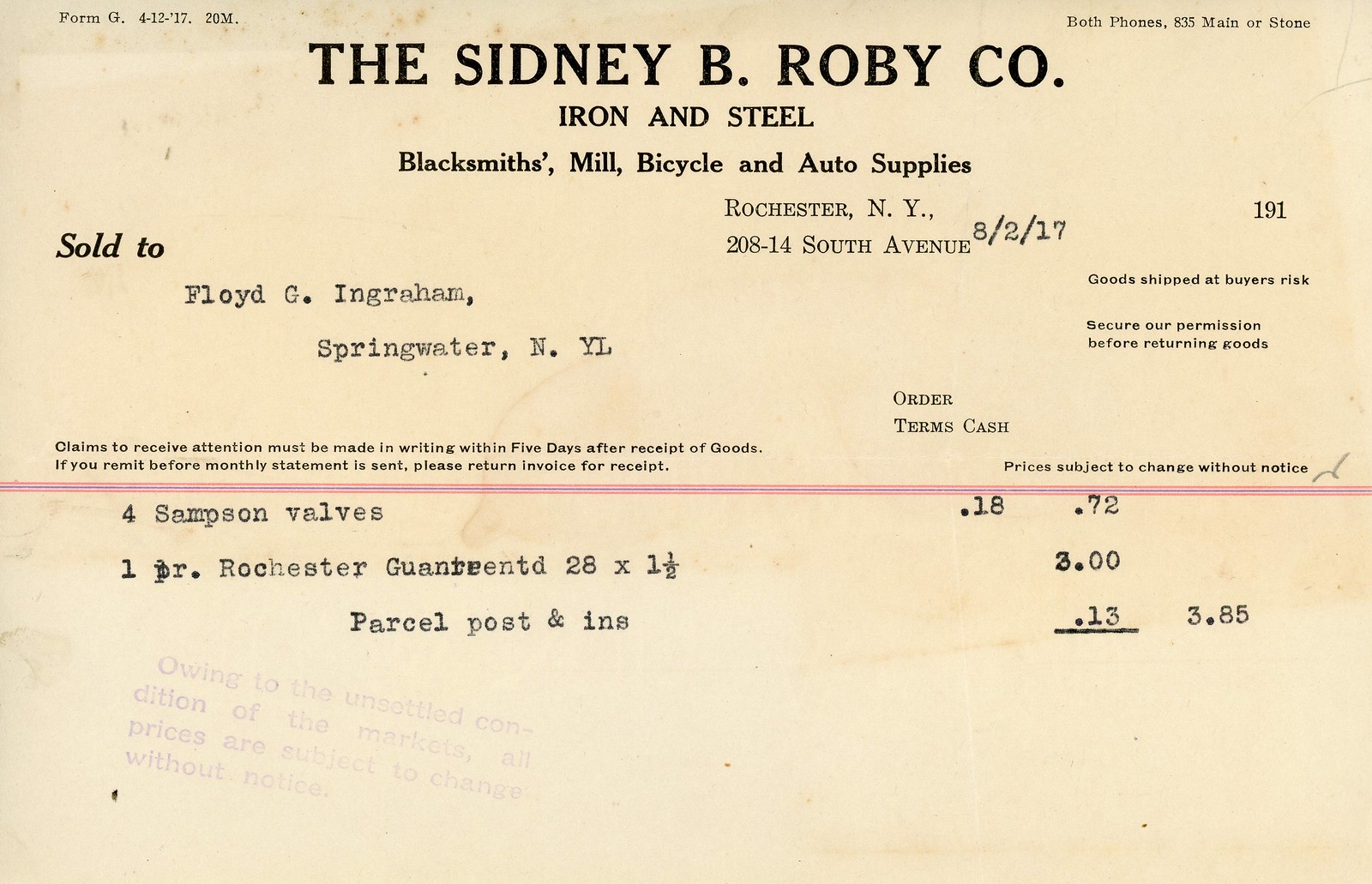This image depicts an old and weathered typewritten receipt on cream-colored cardstock from the Sidney B. Robey Company, based in Rochester, New York, located at 208-14 South Avenue. The header displays the company name prominently, followed by a list of services: iron and steel, blacksmith, mill, bicycle, and auto supplies. The item is dated either August 2, 1917, or potentially 2017, though its aged appearance suggests the former.

The receipt details a purchase by Floyd G. Ingraham from Springwater, New York. The transaction includes four Samson valves priced at 0.18 and 0.72, one PR Rochester guaranteed item at 3.00, parcel post and insurance at 0.13, totaling $3.85. There is a noticeable pink or red horizontal line across the page, with critical notes below it, such as "Owing to the unsettled condition of the markets, all prices are subject to change without notice" and "Goods shipped at buyer's risk. Secure our permission before returning goods. Order terms cash."

In the upper sections of the document, "Form G, 4-12-17-20M" is noted on the left and "Best phones, 835 Maine or Stone" on the right. Another crucial instruction indicates that claims for discrepancies must be made in writing within five days of receipt.